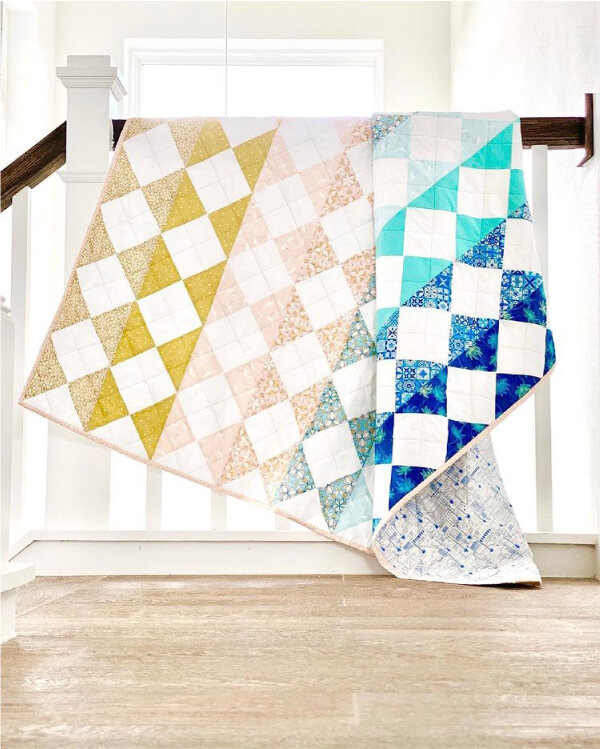This photograph captures a central focal point of a vivid, multicolored quilt hanging on the brown handrail of a stairwell within a house. The stairwell features white vertical pegs supporting the brown railing. The quilt, with its array of colors including yellow, white, blue, pink, and light red, drapes elegantly over the railing. It spans both floors, touching the light hardwood floor in the foreground and cascading over the stairwell in the background. The intricate patterns on the quilt include various checked designs, lending it a dynamic appearance. A window framed in white, along with the white background walls, enhances the quilt's vibrant presence. The overall scene conveys a cozy, warm atmosphere dominated by the striking, elaborate quilt that serves as the photograph's centerpiece.